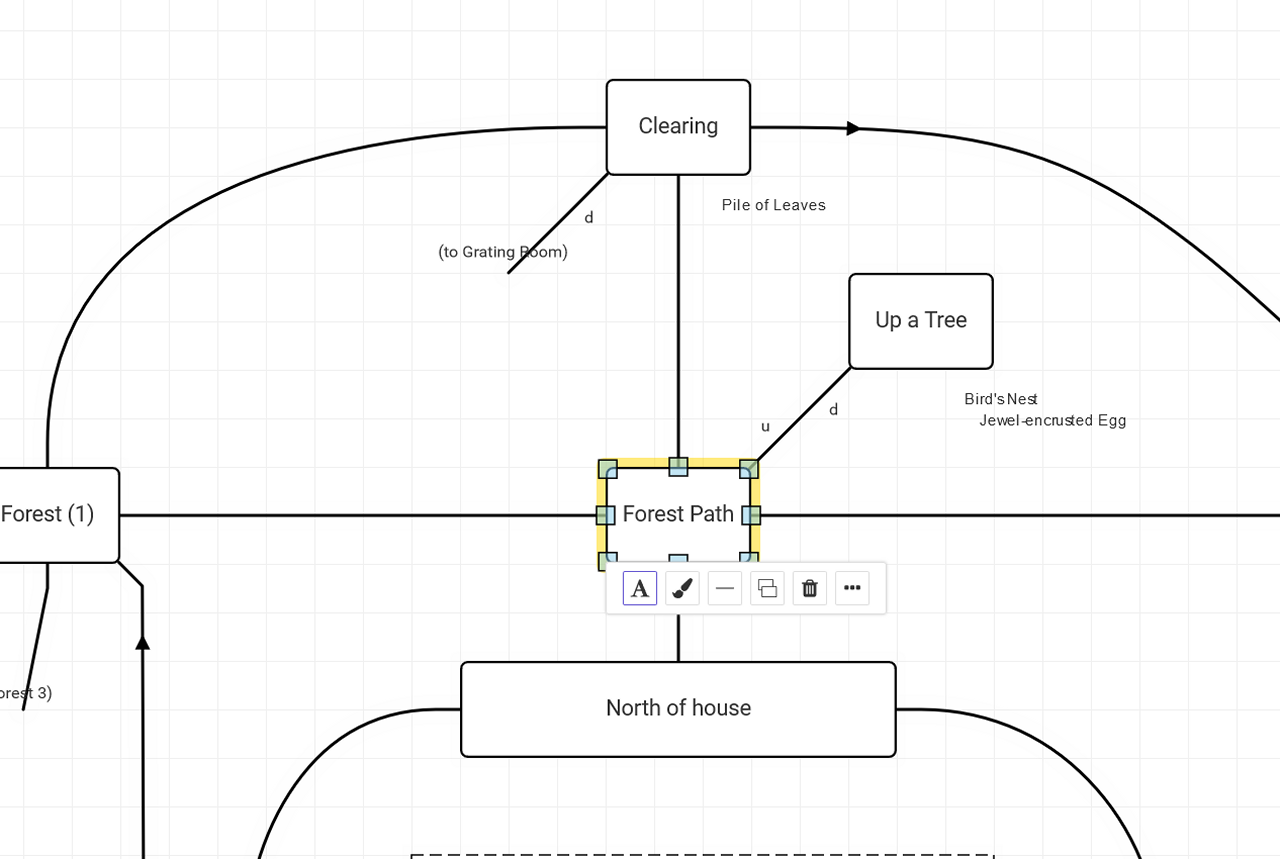The image is a detailed map resembling a video game schematic, rendered on light graph paper. It features various labeled sections connected by thin, penciled-in lines, some highlighted with text boxes. In the center, a yellow, black-bordered box labeled "forest path" is surrounded by smaller green boxes, with black lines connecting it to other parts of the map. Below this central box is a label reading "north of house," suggesting a house just off the visible area to the south. To the left is a section marked "forest," connected by a line downward and labeled with a "1" in parentheses. Above the central box is "clearing," which is connected by a line curving upwards. A text box to the top right-hand corner reads "up a tree," with additional labels "bird's nest" and "jewel-encrusted egg." The map appears monochromatic, except for the highlighted central area, indicating detailed sections and potential pathways within a video game setting.